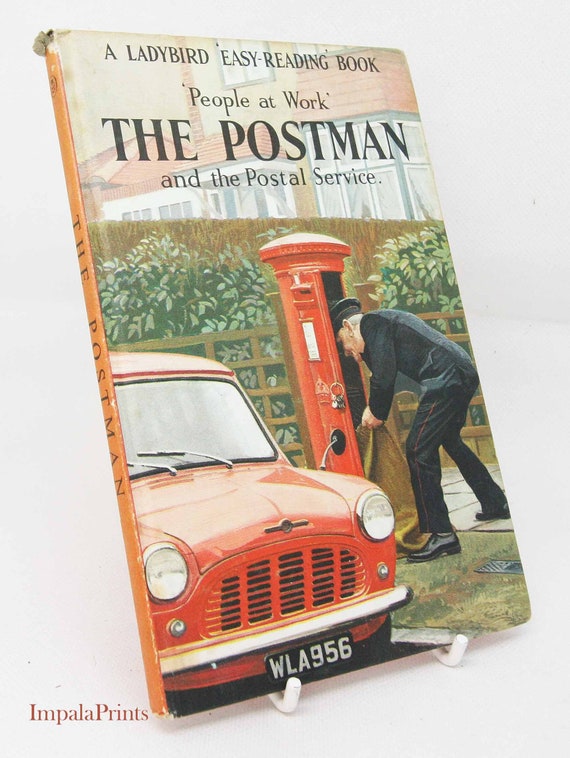This image captures a photograph of a book propped on a white book stand, slightly angled to the right. The title of the book reads "A Ladybird Easy Reading Book, People at Work: The Postman and the Postal Service," with the text styled in varying sizes and boldness. The book's spine is orangish in color, also bearing the title "The Postman." The cover illustration, which appears to be hand-drawn or painted, portrays a scene featuring a man dressed as a postman in a black suit and hat. He is standing on a sidewalk beside a vintage orangish-red car, license plate WLA 956, handling a burlap bag next to a tall, red, cylindrical mailbox with a domed top — presumably collecting mail. In the backdrop, a faintly visible building and a fence blend with some plants, rendering a timeless, almost storybook quality to the scene. The bottom right corner of the image features the text "Impala Prints," indicating the company associated with this presentation. The clean, white background accentuates the detailed cover art of the classic children's book.